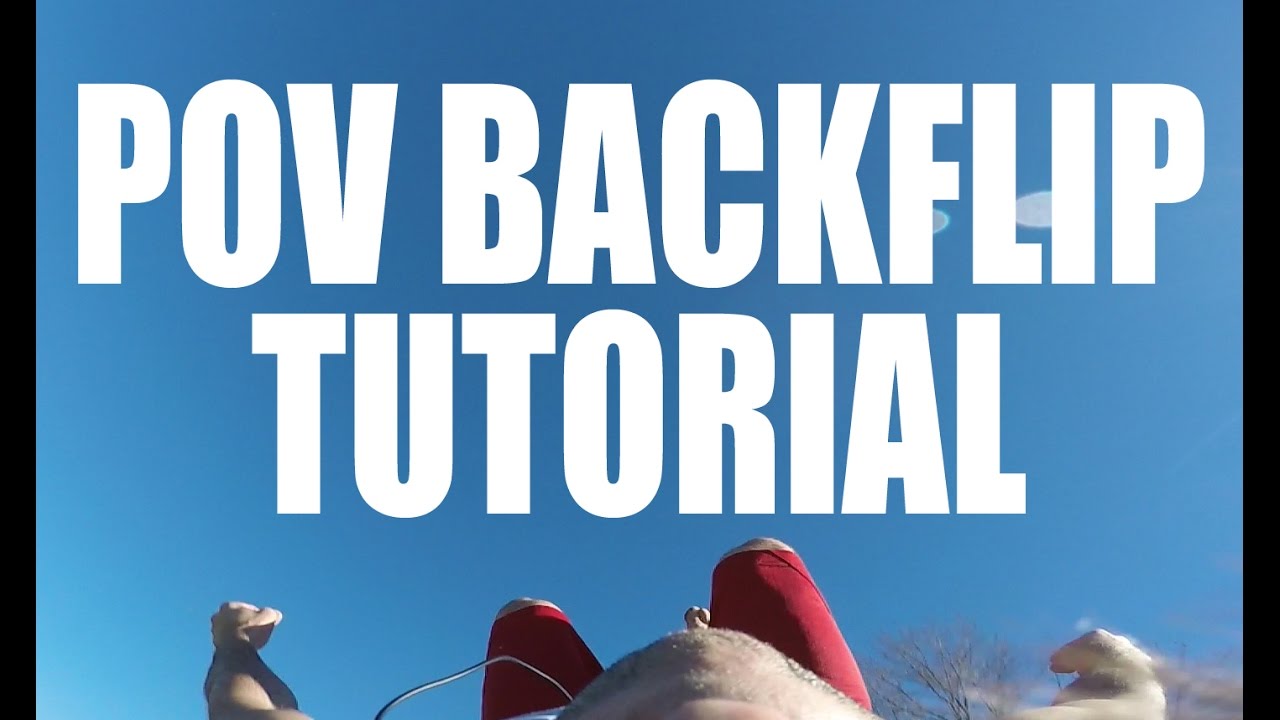This image captures a dynamic moment from a video titled "POV Backflip Tutorial," prominently displayed in large white text over a brilliant blue sky. Framed by two black borders on each side, the scene presents a man mid-backflip, his torso nearly upside down and knees bent above his waist. His arms are outstretched to either side, showcasing muscular definition, while he wears bright red shorts. The lower portion of his head, including his chin and perhaps a bald spot, is visible, adding to the motion-blurred effect of his flip. A small, nearly leafless tree is positioned in the bottom right corner, providing a sense of perspective against the expansive, nearly cloudless sky. Additionally, there appears to be a cable or wire extending from his midsection, adding an intriguing detail to this high-energy instructional moment.